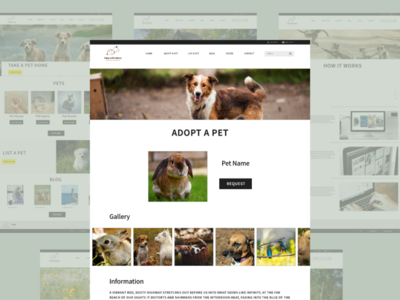**Screenshot Description:**

The image captures a screenshot of a pet adoption website, prominently featuring a central pop-up window that partially obscures the main content. The background displays multiple grayed-out or faded website pages, suggesting a multi-tab interface. The primary color scheme of the background incorporates shades of gray and green, with some discernible sections displaying images of dogs and a labeled section titled "Pets."

On the left side of the faded background, there is a visible picture of a white dog, accompanied by various buttons and options, including a link to the website’s blog. Behind the central pop-up, another website page is slightly visible but largely indiscernible due to the overlay.

To the right of the pop-up, another overlay labeled "How It Works" includes three sections, each featuring cover images such as a computer and a person typing. Further down, two more web pages peek from the bottom of the screen, though they are mostly hidden behind the main pop-up window.

At the center of attention, the bright and clear pop-up window is marked with the title "Adopt a Pet" prominently displayed. The top bar of this pop-up includes a menu with various navigational buttons to different parts of the website and a search bar on the right. The left side of the top bar features the blurred icon of the website, making it difficult to identify the organization.

Inside the pop-up window, a large banner showcases a cover picture of a brown and white dog. Beneath the title "Adopt a Pet," there's an image of a bunny. To the right of this image, there's a section labeled "Pet Name" with a button allowing users to request more information. The lower part of the pop-up includes a gallery section displaying five cut-off images of various pets, such as bunnies, dogs, and birds. Finally, an information icon is situated at the bottom, accompanied by two lines of explanatory text.